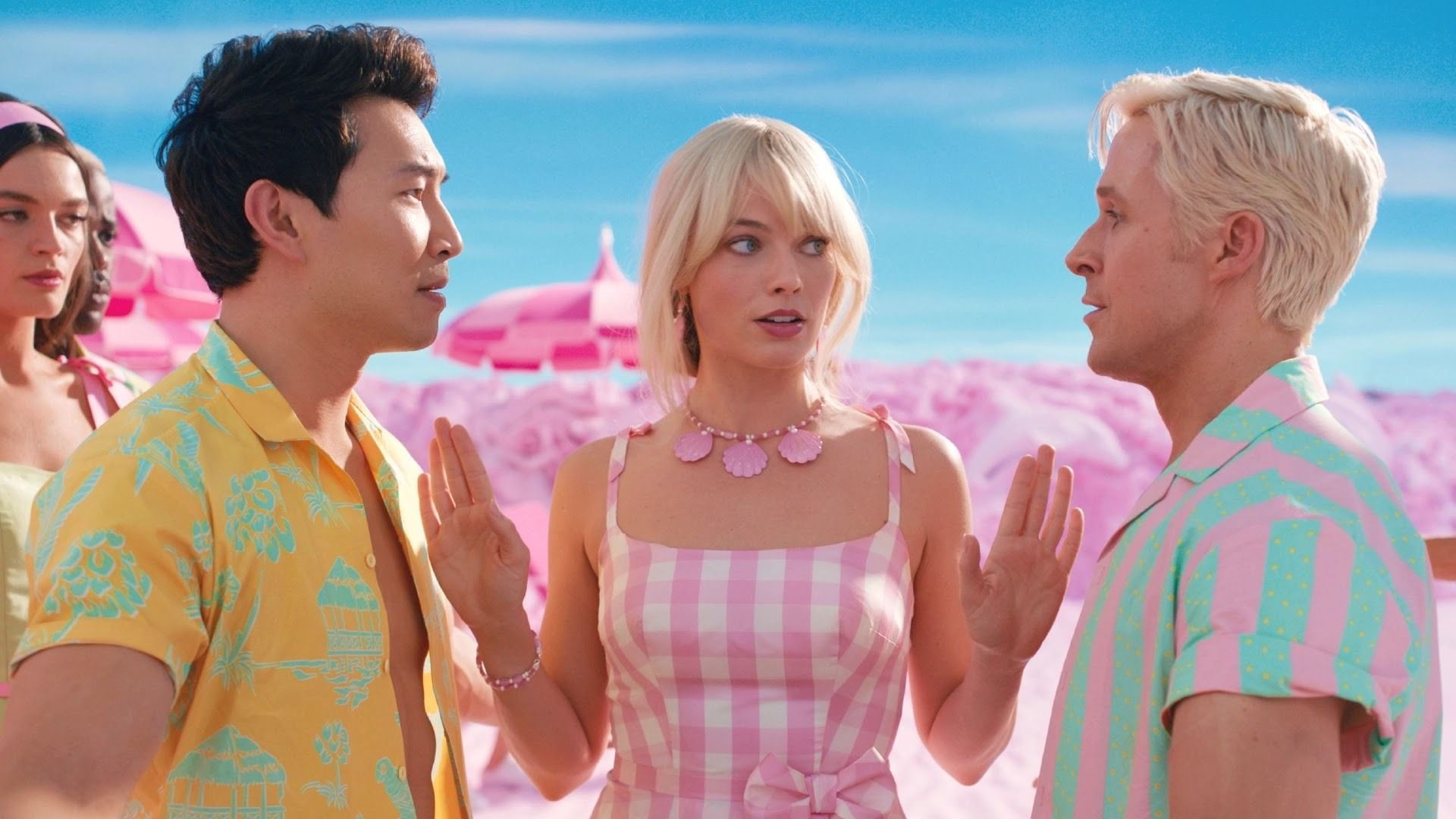In a vibrant scene from the 2023 Barbie movie, Margot Robbie stands in the center as Barbie, with her blonde hair cascading down and a distinctive pink seashell necklace adorning her neck. She is dressed in a sleeveless gingham dress in light pink and white. Flanking her on either side are two men, seemingly in a tense conversation. On her left is Simu Liu, an Asian actor, wearing a yellow short-sleeved Hawaiian shirt adorned with a mint green floral pattern, which is unbuttoned to reveal part of his chest. On her right stands Ryan Gosling, portraying Ken with his bleach-blonde hair, dressed in a short-sleeved button-down shirt featuring vertical stripes in pink, teal, and mint green. Barbie's hands are raised in an attempt to mediate their standoff. Another woman is visible in the distant background standing behind Simu Liu, while pink beach umbrellas dot the scenic backdrop.